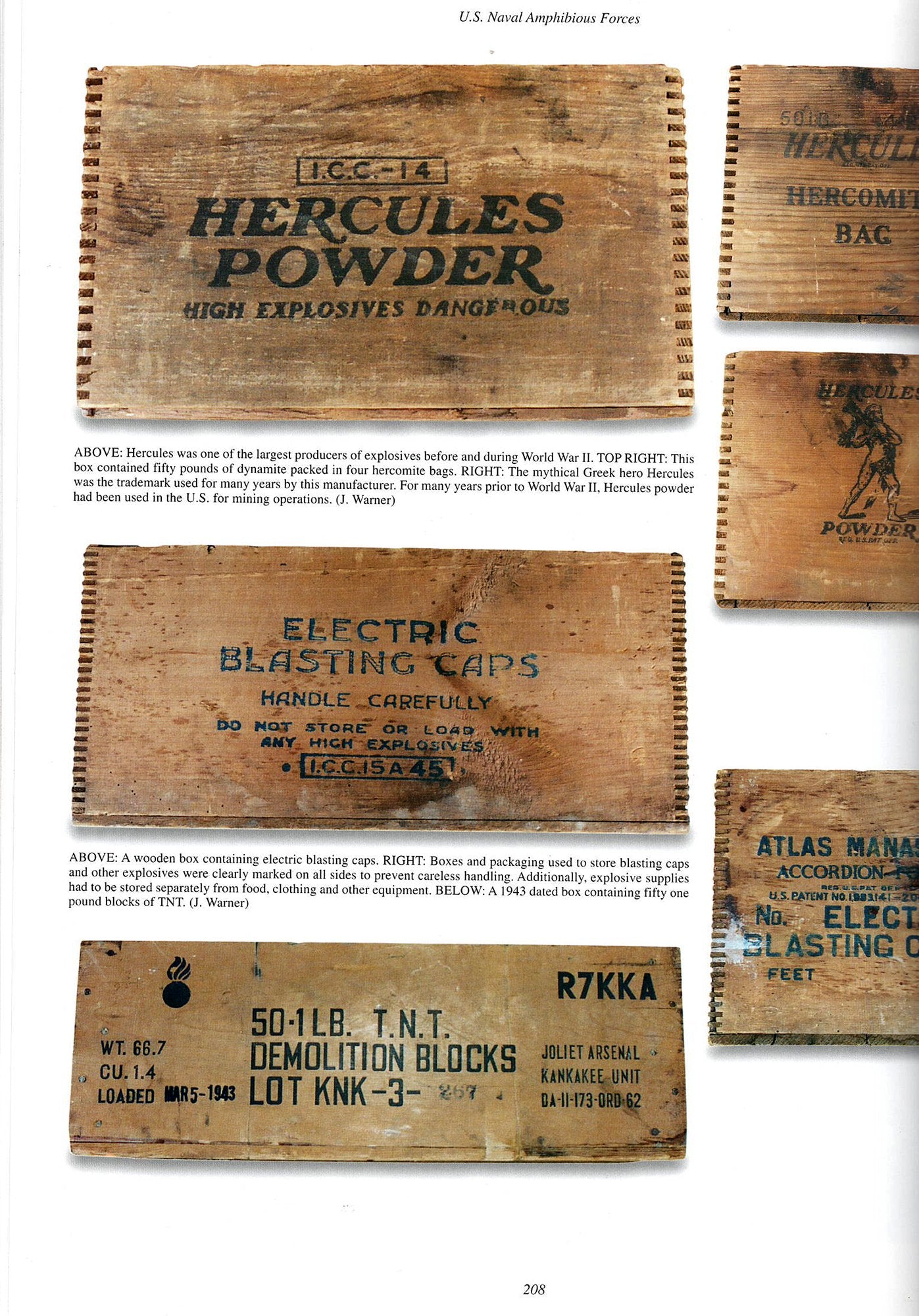This image is a detailed interior page from a book, specifically page 208, featuring six photographic reproductions of wooden crate lids used for storing explosives. The page measures approximately 6 inches high by 4 inches wide, with thin light gray borders on the left and right sides, and a plain white background. At the top of the page, in small black text, it reads "U.S. Naval Amphibious Forces." 

The images on the page include full views of three crate lids on the left and partial views of three more on the right. Each lid displays black printed text detailing the contents and handling instructions. The first crate lid on the top left is marked "Hercules Powder High Explosives Dangerous," accompanied by a paragraph explaining that Hercules was one of the largest producers of explosives before and during World War II, and was also known for its mining operations.

The second lid indicates it contains "Electric Blasting Caps," with a description noting that these caps were packed carefully to avoid being stored with high explosives and must be handled with care. An additional note emphasizes that explosive supplies were always stored separately from food, clothing, and other equipment.

The third lid on the bottom left reads "1943," containing "50-1 Pound Blocks of TNT," including a serial number "R7KKA" and the text "1LB TNT demolition blocks lot KNK-3-." These crates and their markings provide a historical snapshot of explosive storage practices during World War II, underlined by the trademark name Hercules used prior to the war.

At the bottom center of the page, the number "208" confirms this as a specific page from the book, enhancing the context with the detailed descriptions and photographic illustrations.